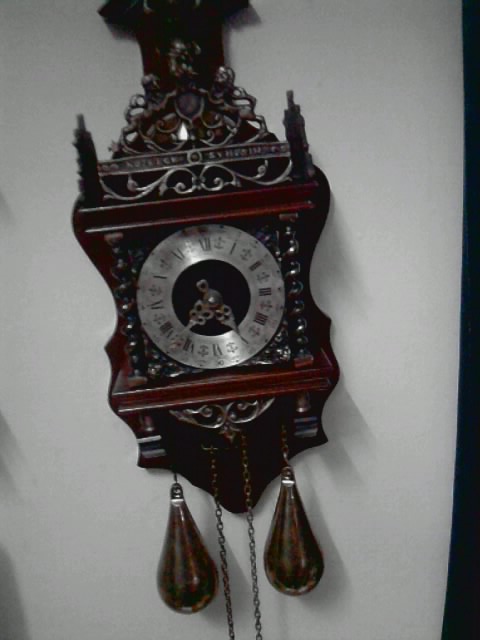The picture captures an intricately designed wall clock hanging slightly askew on a white wall, partly bordered by black on the right. The clock boasts a mahogany wooden body that features a curvy, vertical structure tapering into a neck at the top. A prominent silver coat of arms with two lions is set at the top, flanked by silver scrollwork and an unreadable banner. The clock's wooden supports extend down its sides, meeting two blue columns accented by silver markings resembling leaves, along with additional decorative metal pieces. Its face is adorned with black Roman numerals on a silver background, and features mahogany hands with unique circular designs suggesting the time is around 5:36. Two long chains hang from the clock, paired with large, brass teardrop-shaped weights that could chime the hours. The clock's overall elaborate and decorative elements make it a distinctive and detailed timepiece.